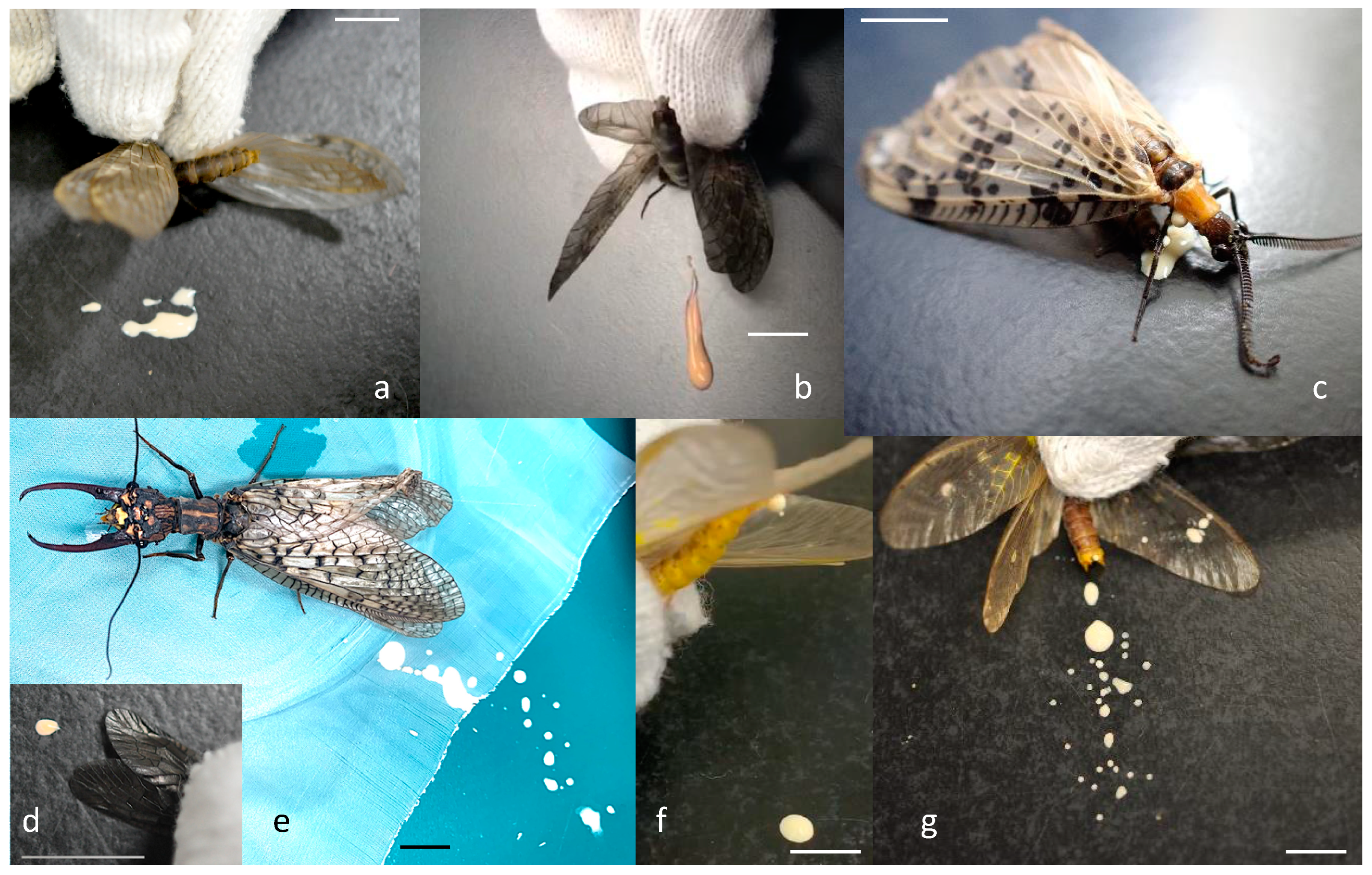The image comprises a series of pictures depicting interactions with a Dobson fly. In the upper left (Image A), a man wearing white gloves is pressing on the Dobson fly, causing a white liquid to emerge. Moving to the top middle (Image B), the fly is again being firmly held by the gloved hand, releasing an orange liquid. The upper right (Image C) shows the Dobson fly resting on a black surface, revealing its cream-colored wings with black spots, an orange body, and a burgundy head with black legs and antennae. The lower left (Image D) presents a close-up of the fly's black wings. Above this, in the middle left (Image E), the Dobson fly sits on a blue surface, displaying large pinchers on its face, with a black body, head, legs, and antennae. The wings here are beige with black spots. To the right (Image F), the fly's wings are shown being held by white gloves, exposing an orange segment of its body beneath. Finally, in the bottom right (Image G), the fly, grasped by white gloves again, squirts out a yellowish liquid.